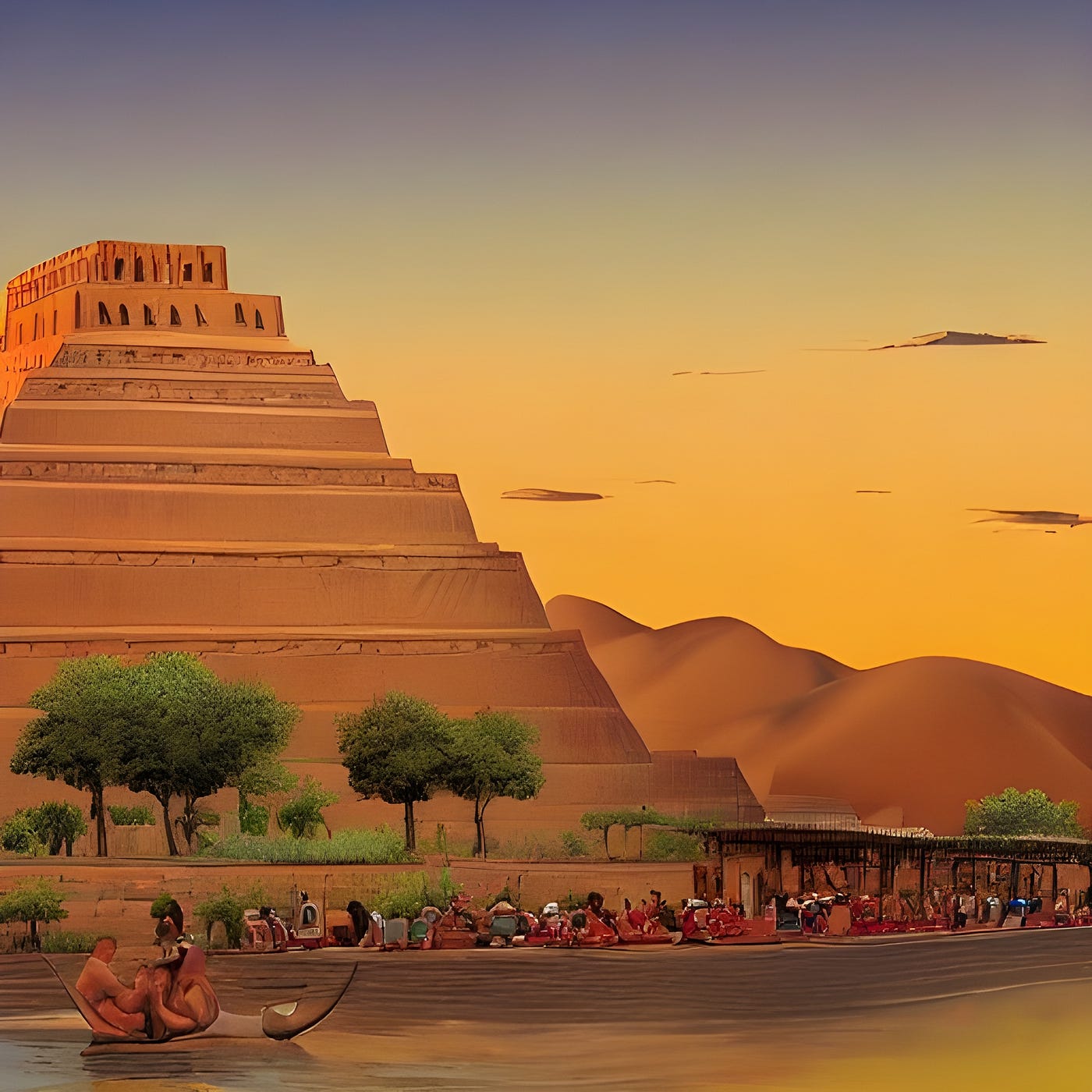The image depicts a surreal, possibly AI-generated landscape dominated by an unusual pyramid situated on the left side. The pyramid appears to be of Aztec or Egyptian inspiration and is constructed from goldish-yellow to brownstone. Its distinctive shape features a flat summit, crowned by a small sandstone structure with black windows. The pyramid is tiered with at least eight layers, each smaller than the one beneath it. In the foreground, a river occupies the lower part of the scene. On the far bottom left in the water, a poorly rendered boat with two misshapen, almost grotesque human figures adds an eerie touch. The riverside is crowded with an indistinct crowd of people in colorful clothing, seated alongside trees and bushes, with some taking shelter under a roofed area on the right. Beyond the river, rolling golden-brown hills form the background, all bathed in the warm hues of an orange sunset, which transitions to a bluish sky above.